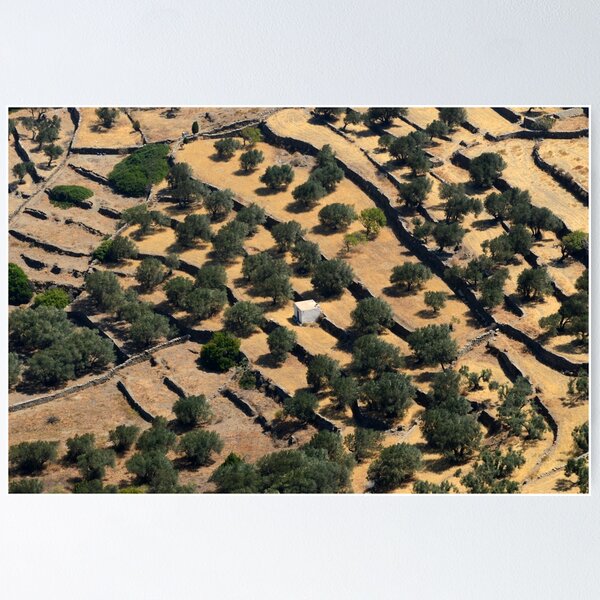The image appears to be an aerial photograph of a dry, parched landscape characterized by a maze-like arrangement of staggered fencing or stone walls that zigzag across the terrain. In the center of the photograph stands a tall, white box-shaped building, possibly a house or storage structure. Surrounding this lone building are numerous small, round green trees and bushes. The ground between these vegetation clusters is barren and brown, showing no signs of lush greenery. There are also dark trails crisscrossing the land, which could be paths or driveways. The entire scene feels deserted, with no visible people, animals, or other buildings, giving an impression of isolation amid the meticulously sectioned landscape.